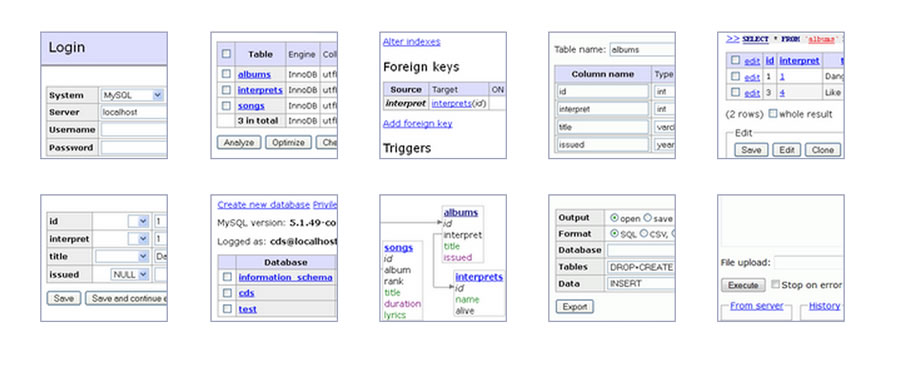This is a detailed screenshot of a web page displaying 10 distinct information boxes arranged side by side. Each box contains various pieces of information and action buttons, accentuated with a color scheme of black and white, interspersed with blue, green, purple, and a touch of red text.

1. The first box lists essential login details such as "Login, System, Server, Username, Password."
2. The second box pertains to tables with blue-highlighted categories like "Albums, Interprets, Songs," and includes action buttons labeled "Analyze" and "Optimize."
3. The third box focuses on foreign keys and concludes with a mention of "Triggers" at its bottom.
4. The fourth box is centered around database tables with identifiers such as "Table Name: Albums" followed by a list of column names.
5. The fifth box features selection options with various "Edit" buttons and functions like "Save," "Edit," and "Clone."
6. The first box on the bottom row includes fields labeled "ID, Interpret, Title Issued" along with drop-down menus and buttons labeled "Save" and "Save and Continue."
7. The second box on this row is for database creation, containing options titled "Create New Database" with categories like "Information Schema, CDs, and Tests."
8. The third box lists musical components "Albums, Songs, Interprets."
9. The fourth box outlines export settings with entries like "Output Format, Database, Tables, Date" followed by an "Export" button.
10. The final box on this row deals with file uploads, featuring an "Execute" button along with a "Stop on Error" option.

This organized layout suggests a user interface designed for database management or development, providing various functional tools and navigation options for efficient data handling and manipulation.